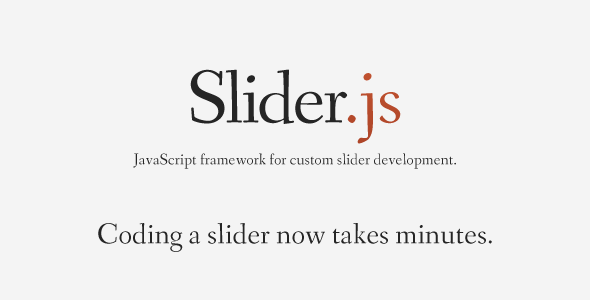The image features a promotional graphic for "Slider.js" displayed within a rectangular box set against a light gray background. The box has a somewhat unique shape, resembling a "fatter" rectangle—not quite the elongated form typically seen, yet also not square.

The text within the rectangle maintains a censored appearance, all characters being black except for one stylish detail. The font mimics the look of an old-school typewriter. The term "Slider.js" is prominently displayed, with "Slider" in black while the ".js" suffix is in red, providing a stark contrast.

Directly below, a subtitle reads, "JavaScript Framework for Custom Slider Development." This is followed by a noticeable triple space. The final line concludes with the statement, "Coding a Slider Now Takes Minutes," suggesting significant practicality and efficiency improvements, pointing towards an advertisement.

No additional branding or logos are present to further clarify, but the phrasing indicates a commercial intent, implying recent updates or enhancements have made slider coding substantially quicker.